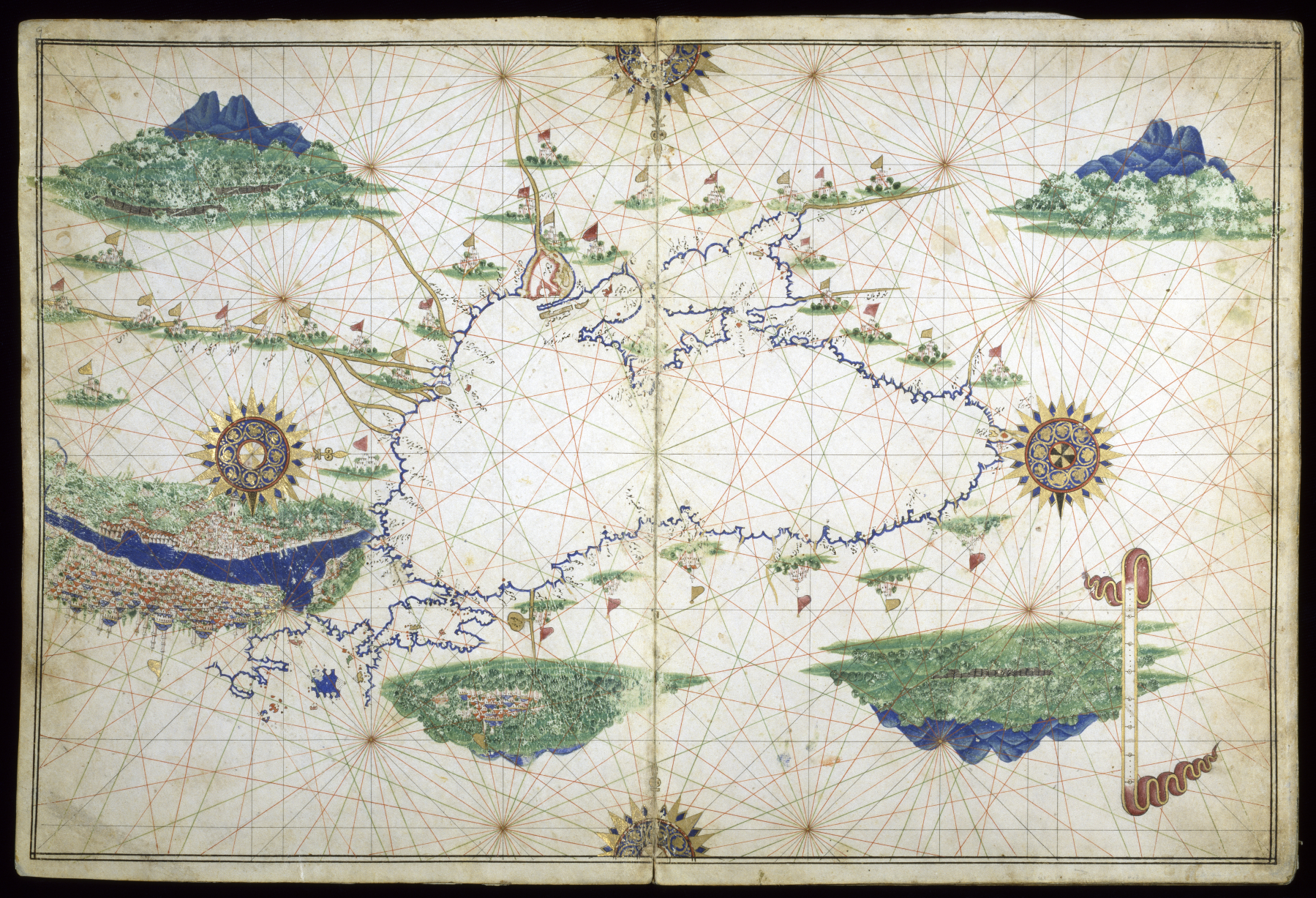This colorful and slightly landscape-oriented photograph captures an ancient, well-worn map set against an ivory background marked by the unmistakable signs of aging, including pronounced creases, smudging, and feathering in shades of gray and brown. Unfolded from a previous state of being halved, the map delineates several distinctly illustrated territories, predominantly bordered in blue. The central feature is a bold blue outline of an undefined land or body of water. This map displays a total of five prominent land masses placed in various positions: one in each upper corner, one in the left middle, one prominently in the center, and another in the right corner. Each land mass is adorned with intricate illustrations of blue mountains atop green vegetation, evoking a sense of lush, yet mysterious, geography.

Distributed across the map are multiple notable symbols, including 29 small flag markers on the different geographical features, suggesting significant points or landmarks. Four stars with radiating rays mark the cardinal directions, enhancing the navigational aspect of the map. The land masses in the lower half appear uniquely reversed, with mountains oriented upside down. Additionally, light golden lines crisscross the map, potentially indicating pathways, distances, or other navigational aids. The corners and borders of this historical artifact feature scenes of mountain landscapes and greenery, and in the lower right corner, a snake-like creature adds an element of mythical intrigue. The primary colors of this map—blue, green, and gold—stand out vividly against its timeworn canvas.